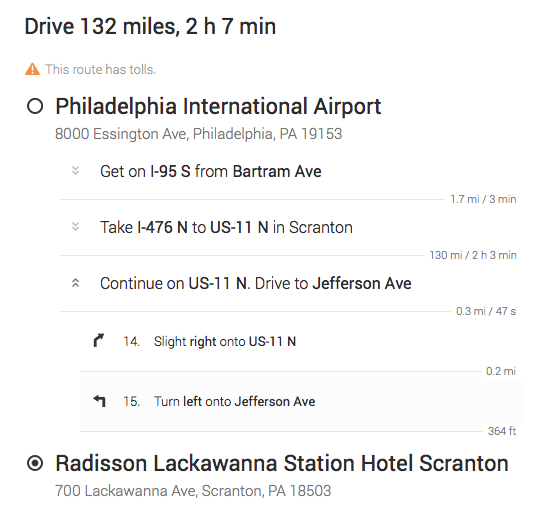This image features detailed driving instructions from Philadelphia International Airport to the Radisson Lackawanna Station Hotel in Scranton, Pennsylvania. The directions, displayed in black text on a white background, indicate a total journey of 132 miles, estimated to take two hours and seven minutes. Starting at the Philadelphia International Airport, located at 8000 Essington Avenue, Philadelphia, PA 19153, the instructions begin with getting on I-95 South from Bartram Avenue for a distance of 1.7 miles, which should take three minutes. 

The next leg of the journey involves taking I-476 North to US 11 North in Scranton, covering 130 miles in about two hours and three minutes. Upon reaching Scranton, the directions advise continuing on US 11 North, then driving 0.3 miles to Jefferson Avenue. Specifically, you'll need to take a slight right onto US 11 North, continue for 0.2 miles, and then make a left turn onto Jefferson Avenue for 364 feet to reach your destination. The instructions also highlight that this route includes tolls, marked with a yellow triangle containing an exclamation point. The final destination is the Radisson Lackawanna Station Hotel at 700 Lackawanna Avenue, Scranton, PA 18503.